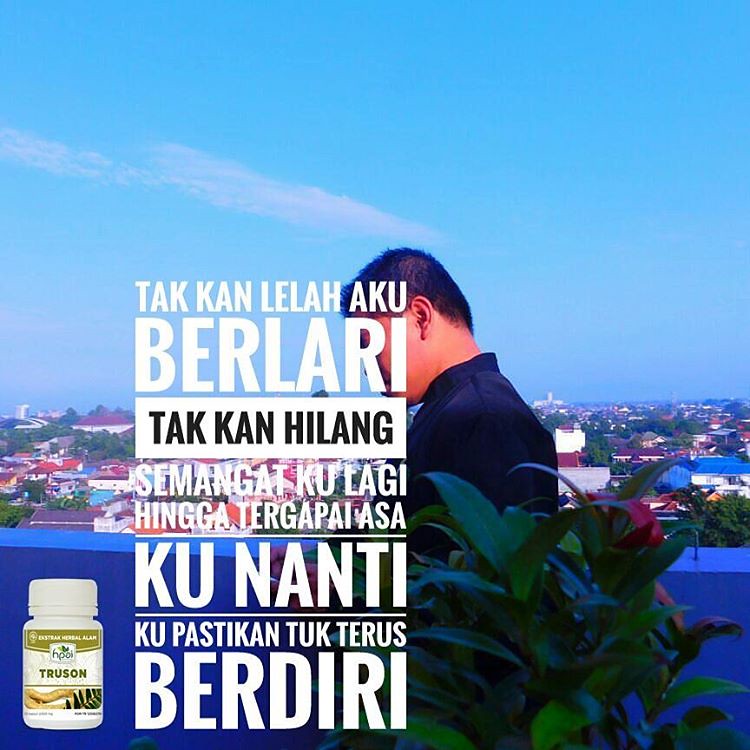In this outdoor advertisement, a man, possibly Asian, stands on a balcony or rooftop facing left. He is wearing a purple shirt and has short black hair. However, his face is obscured by white and black text, with phrases in a foreign language such as "Takkan Leila aku burlari" and "semigod koolagi hinga Turk Turgapai asa." The text also includes a brand name, "trucent," near a bottle depicted in the bottom left corner, suggesting the ad promotes an herbal medicine or supplement. The scene features a partly cloudy sky with blue hues, a distant town with modest buildings, and what might be a silo far away. In the foreground to the right, there's a green bush, likely real, as it adds to the natural setting of the image. The overall colors in the advertisement are blue, green, white, and black.